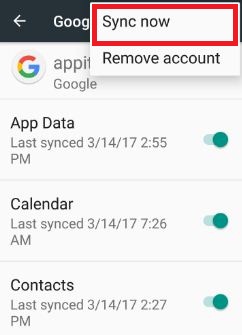The screenshot displays a section of the Google account synchronization settings on a device. The top bar of the screen is navy blue and features a white, left-facing arrow for navigation, along with the word "Google." A red rectangle frames the top part of the screenshot, drawing attention to two options: "Sync now" and "Remove account." Below this section, the Google icon is prominent. The subsequent content lists various types of data with their last synchronization times and corresponding toggles, all highlighted in green to indicate active syncing. Specifically, "App data" was last synced on March 14, 2017, at 2:55 PM; "Calendar" was last synced on the same day at 7:26 AM; and "Contacts" was last synced at 2:27 PM on March 14, 2017. All three data categories have enabled toggles, signifying they are set to sync automatically.